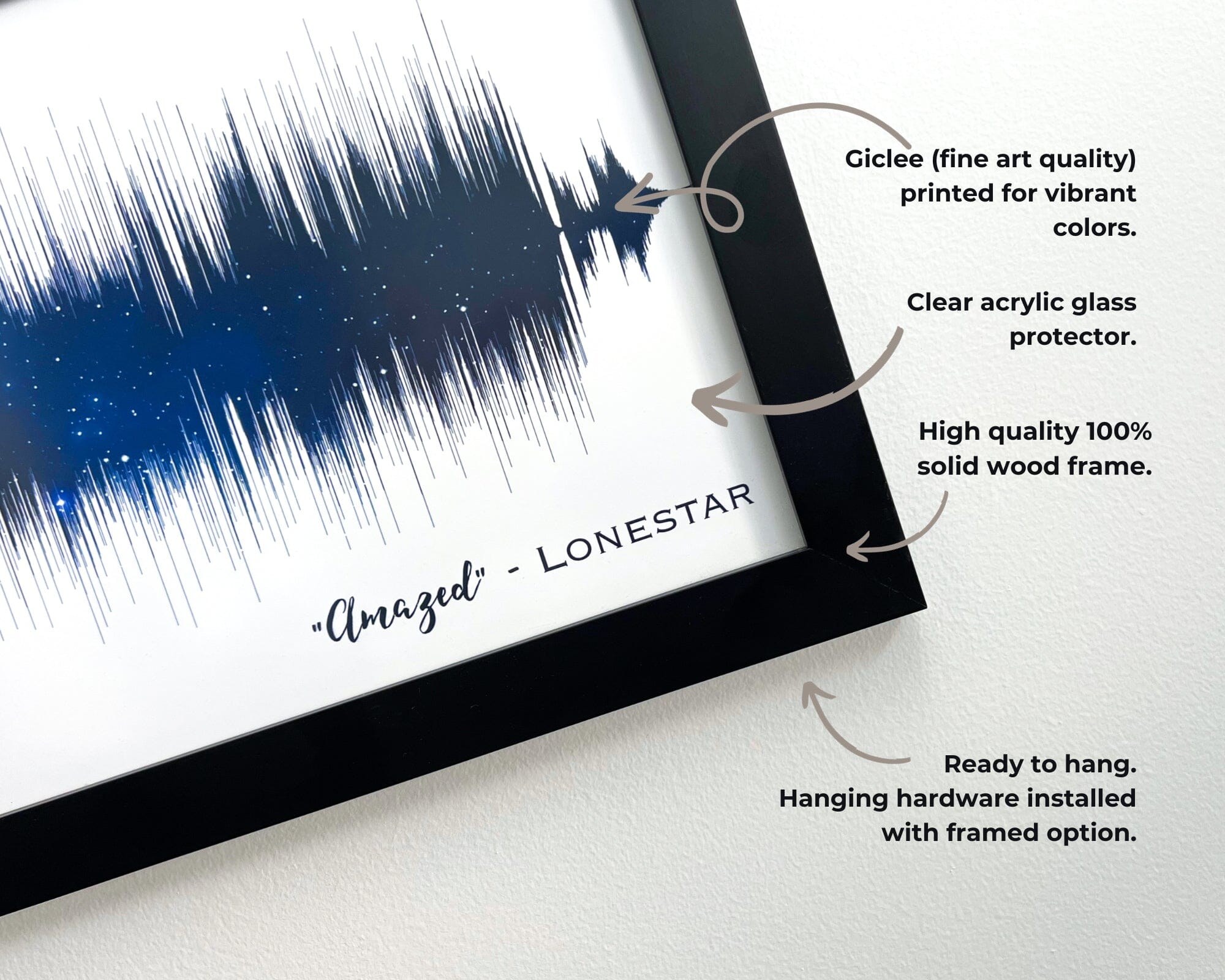This image is an advertisement for a piece of artwork that is displayed in a high-quality black picture frame. The centerpiece of the artwork features a visual representation of a sound wave, commonly seen when mixing audio, overlaying a clean white background. The vibrant blue sound wave is adorned with white specks, adding a dynamic element to the piece. Beneath the sound wave, the phrase "amazed" is written in an italic, funky font, followed by "- Lone Star" in a bold font, suggesting that the sound wave may represent a song by that name. 

The frame is depicted at a slight angle, and several arrows on the image point to different features, explaining the product’s specifications. One arrow points to the sound wave and reads, "Geekly, fine art quality, printed for vibrant colors." Another arrow highlights the frame’s clear acrylic glass protector. Additional text points to the frame itself, noting its "high quality, 100% solid wood frame." The frame comes "ready to hang" with hanging hardware already installed, making it convenient for immediate display. The background around the frame resembles a light white wall texture, further emphasizing the artwork's modern and clean design.